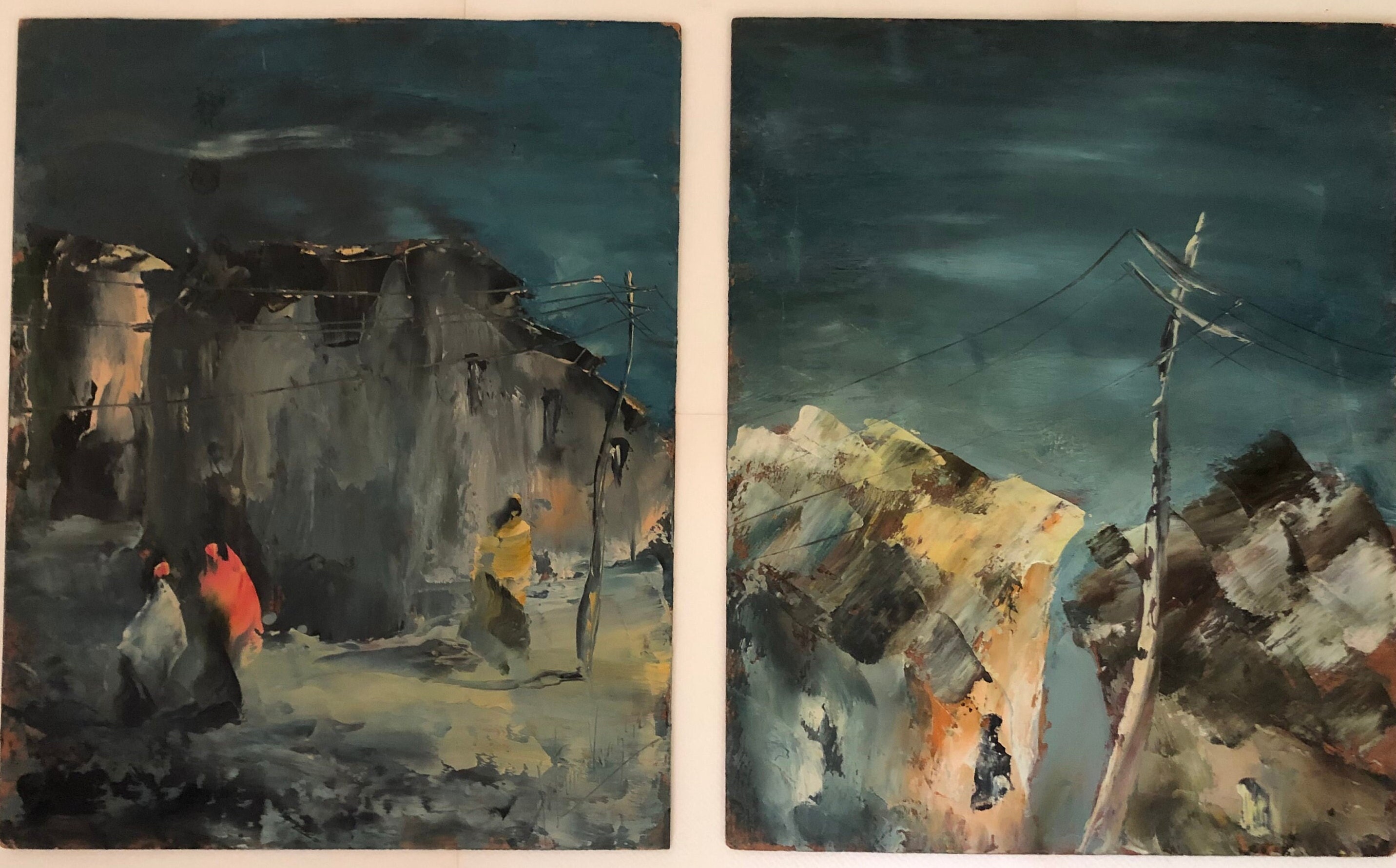The image showcases two side-by-side, oil-based paintings, likely created by the same artist due to their cohesive style and color palette. Both paintings exude a dark and gloomy atmosphere, employing a combination of dark blues, grays, browns, and blacks. On the left, the painting features a moody sky over a rugged, rocky landscape with a slightly wavy utility pole and telephone wires overhead. Below, three abstract figures stand; one is in red, another in white, and the third in black, with a fourth figure in a yellow dress slightly further away. The ground in this image has a bluish-gray hue, blending seamlessly with the figures and surroundings. The image on the right mirrors this dark, craggy setting with two large rocks flanking a central, distorted utility pole. Here, no figures are present, but the continuity of the power line and the similar use of color suggest a thematic or narrative link between the two works. Together, these paintings create a haunting, surreal landscape that feels part of a larger, cohesive composition.